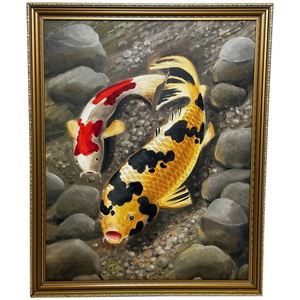This image is a framed artwork, taller than it is wide, featuring two koi fish amidst a rocky background. The frame is a simple yet shiny gold color, rectangular in shape. The backdrop consists of a gray bed scattered with tiny pebbles, and larger rocks are arranged on both the right and left sides. At the very center of the composition is a large, gold-colored koi fish adorned with black spots. To the left of this fish is a slightly smaller white koi with prominent red spots. This detailed and colorful depiction brings the serene underwater scene to life.